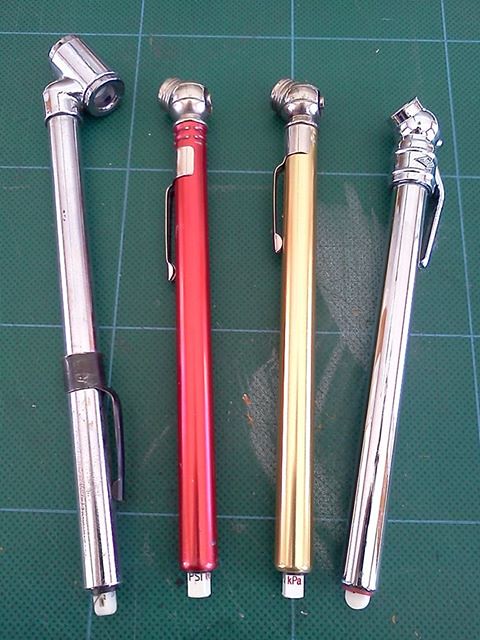This image displays four tire pressure gauges arranged side by side on a surface with green, dirty plaid-like tiles and blue grid lines. The gauges have a metallic reflective coating with varied colors: the leftmost one is silver, followed by red, gold, and another silver. All four gauges are pen-like in shape with white tips at the bottom, which have legible lettering specifying units like PSI and KPA to measure tire pressure. The gauges feature clips, similar to those on pens, allowing for easy attachment to pockets. Each has a ball-shaped figure at the top end, contributing to their distinctive design.